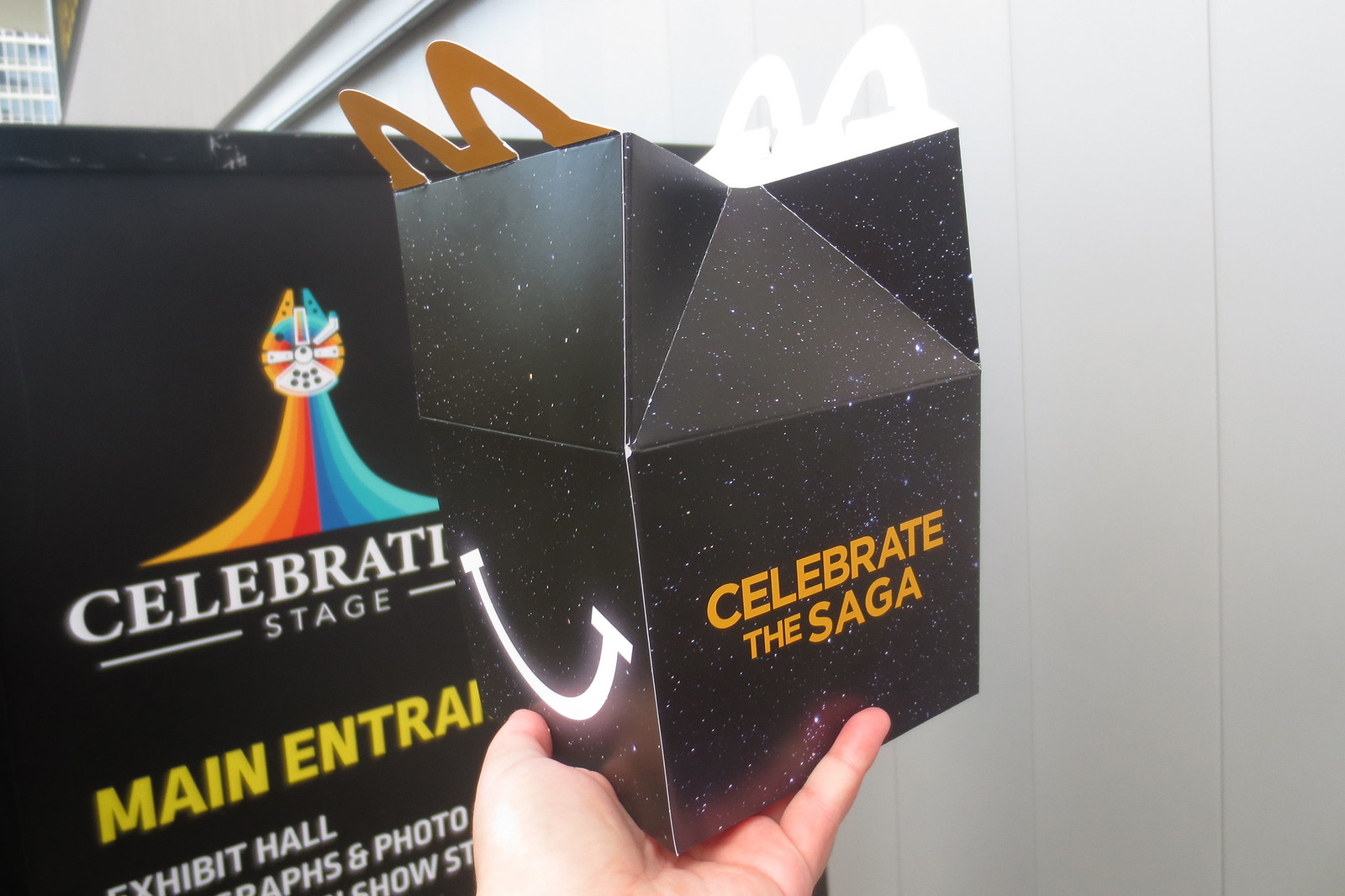In this image, a person is holding an open special edition McDonald's Happy Meal box in their left hand. The box is distinctively black with white star-like spots, evoking a galaxy theme. On one side of the box, a white stylized smile is prominently displayed, while the other side features yellow text that reads "Celebrate the Saga." The characteristic folded top of the Happy Meal box is open. The backdrop consists of a solid gray wall with a black banner. The banner is emblazoned with the text, "Celebration Stage, Main Entrance, Exhibit Hall, Graphs and Photo," hinting at an event or convention. Above the banner's text, a vibrant image of the Millennium Falcon from Star Wars is depicted, launching upward with a colorful rainbow trail that includes shades of yellow, orange, red, and blue, adding to the celebratory atmosphere of what appears to be a Star Wars-themed event.